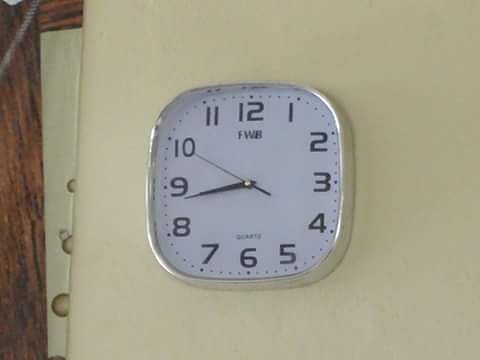The image features a unique clock with a mix of square and circular shapes, boasting curved corners and a prominent silver metal edge. The clock has a white face with bold black hands and numerals, showing the time as 8:44, with the second hand positioned at the 50-second mark. It also displays the label 'FWR' at the top and 'Quartz' above the 6 o'clock position. The background includes a light tan or yellowish wall where the clock is mounted, along with hints of a picture frame and a wooden door frame. Additionally, the clock face features small dots between the numbers to indicate seconds, providing precise time indication.